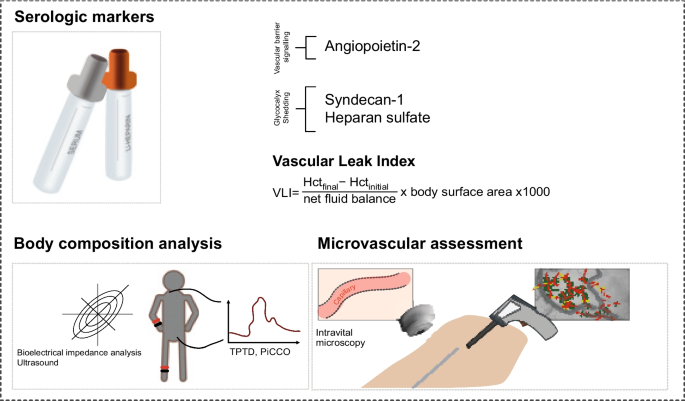The image, likely from an educational or medical textbook, features a detailed instructional layout divided into three main sections outlined by a black dotted rectangular frame on a white background. In the top left corner, there is a section labeled "Serologic Markers," which depicts two small transparent vials, one with a red cap and the other with a gray cap, representing blood sample collection tools.

Below this, in the bottom left portion, a segment titled "Body Composition Analysis" presents an intricate image within a rectangular box. This illustration includes a human figure marked with red and black bands around the wrists and ankles, accompanied by a radar-like logo indicating techniques such as bioelectrical impedance analysis and ultrasound. There's also a sinusoidal graph labeled with terms like PPTD and PICCO, signifying various body composition metrics.

On the right side, a section labeled "Microvascular Assessment" features a detailed image of an arm undergoing some sort of medical procedure, possibly involving a specialized tool for extracting or analyzing tissue. This area also includes smaller images highlighting body tissues and is annotated with terms like intravital microscopy and vascular leak index. Additionally, there are equations and terms associated with vascular barrier signaling, such as angiopoietin 2, glycocalyx shedding, syndecan 1, and heparan sulfate, indicating a deep focus on microvascular health.

Overall, the image serves as a comprehensive instructional reference, integrating various elements crucial for understanding serologic markers, body composition analysis, and microvascular assessment.